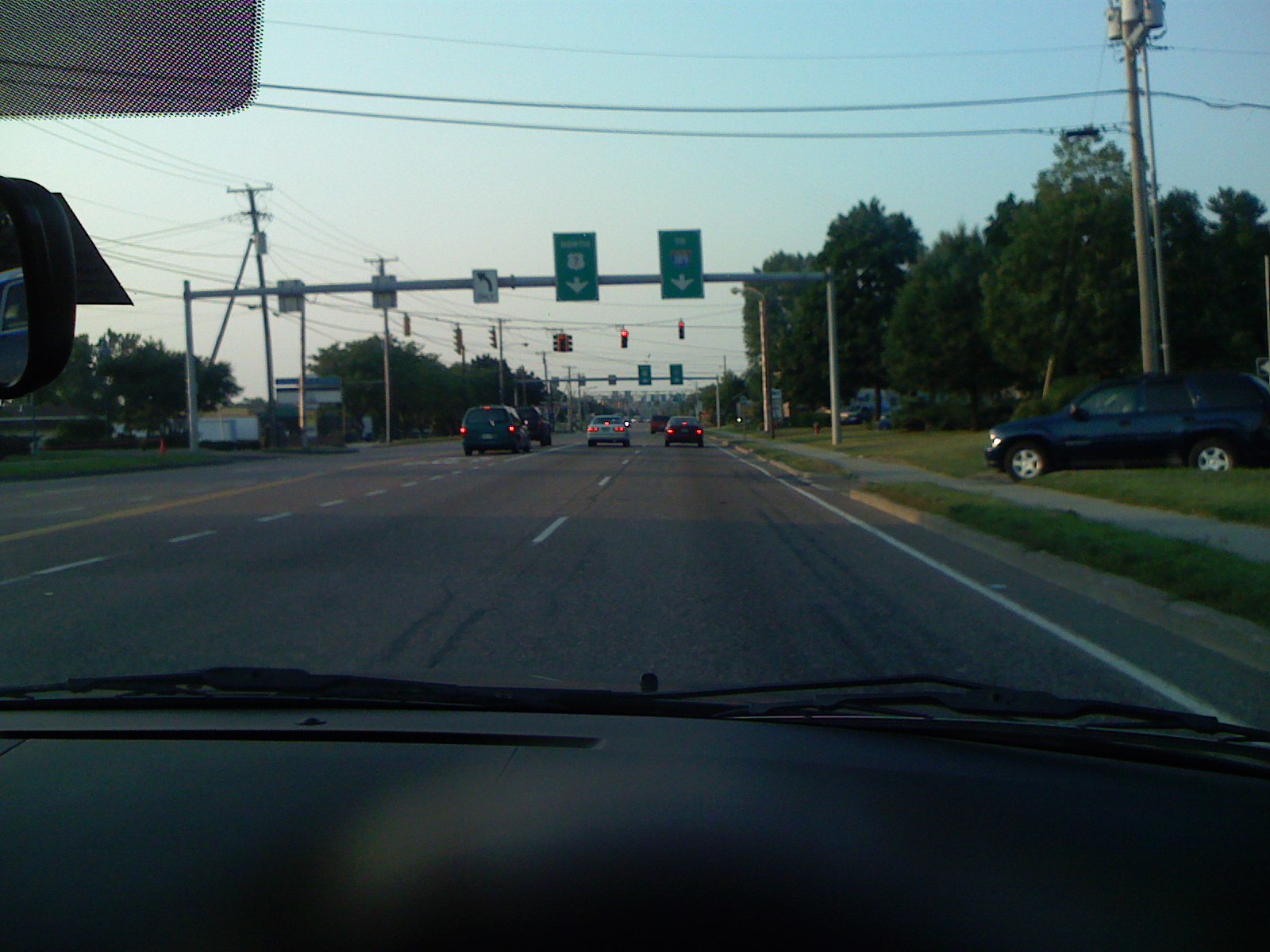This image captures a late afternoon scene of traffic from a driver's viewpoint. In front of the driver, there are four cars stopped at a red traffic light: two minivans in the left lane, a white sedan in the middle lane, and a dark-colored car in the right lane. To the right side of the road, a grass strip and a sidewalk are visible, along with a dark blue-black SUV that appears to be either parked or pulling out. The driver’s black dashboard and partially seen visor with a small mirror are in view at the top of the image. On the left side of the road, a gas station or building with a billboard can be seen, though it is slightly unclear. A route sign indicating "345" and a "North 7" sign are clearly visible, along with a left turn signal and white road striping. Additional parked cars are also visible, completing the scene.